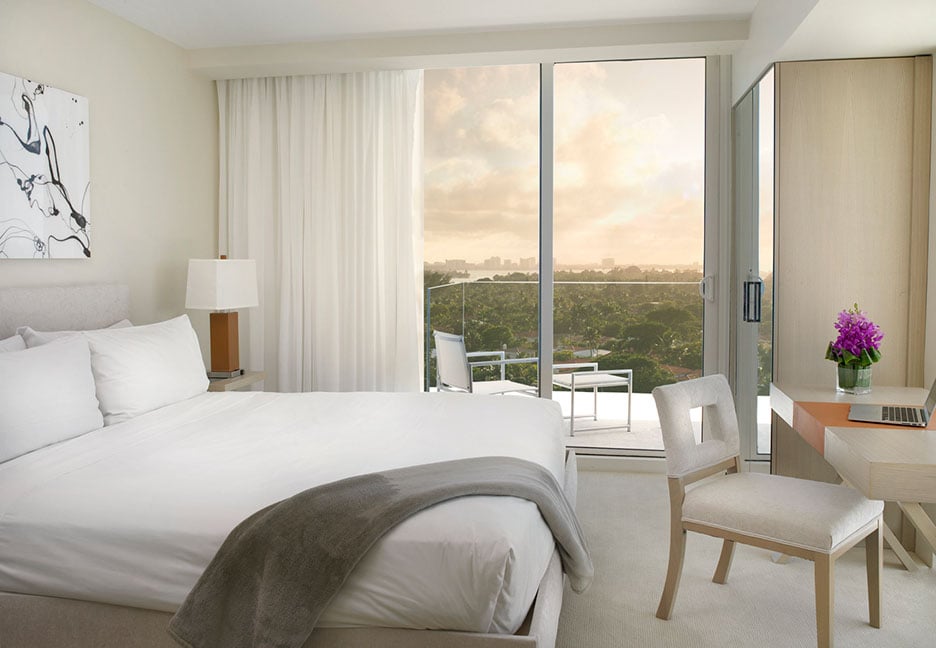The photograph captures a crisp and neatly organized hotel room with predominantly white decor. On the left side of the image and extending toward the center, a queen-sized bed is draped in white sheets and topped with two white pillows. A gray or blue blanket hangs off the corner of the bed. Above the bed, a striking painting with abstract white and black splatters adorns the wall. Adjacent to the bed, on its left, a small nightstand stands with a lamp on it.

To the right of the bed is a modern chair featuring white cushions and wooden legs, pulled out slightly from a floating desk. This white and brown desk supports an open silver laptop and a purplish flower in a small pot, adding a hint of color to the room. The desk is positioned near a closet with mirrored or glass doors.

Further to the right, in the middle of the background, large white curtains frame a sliding glass door that leads to a balcony. This balcony offers a view of a lush park filled with green trees, with buildings peeking through in the distance. The sky above encapsulates a serene palette of peach, light blue, and white hues, sprinkled with clouds.